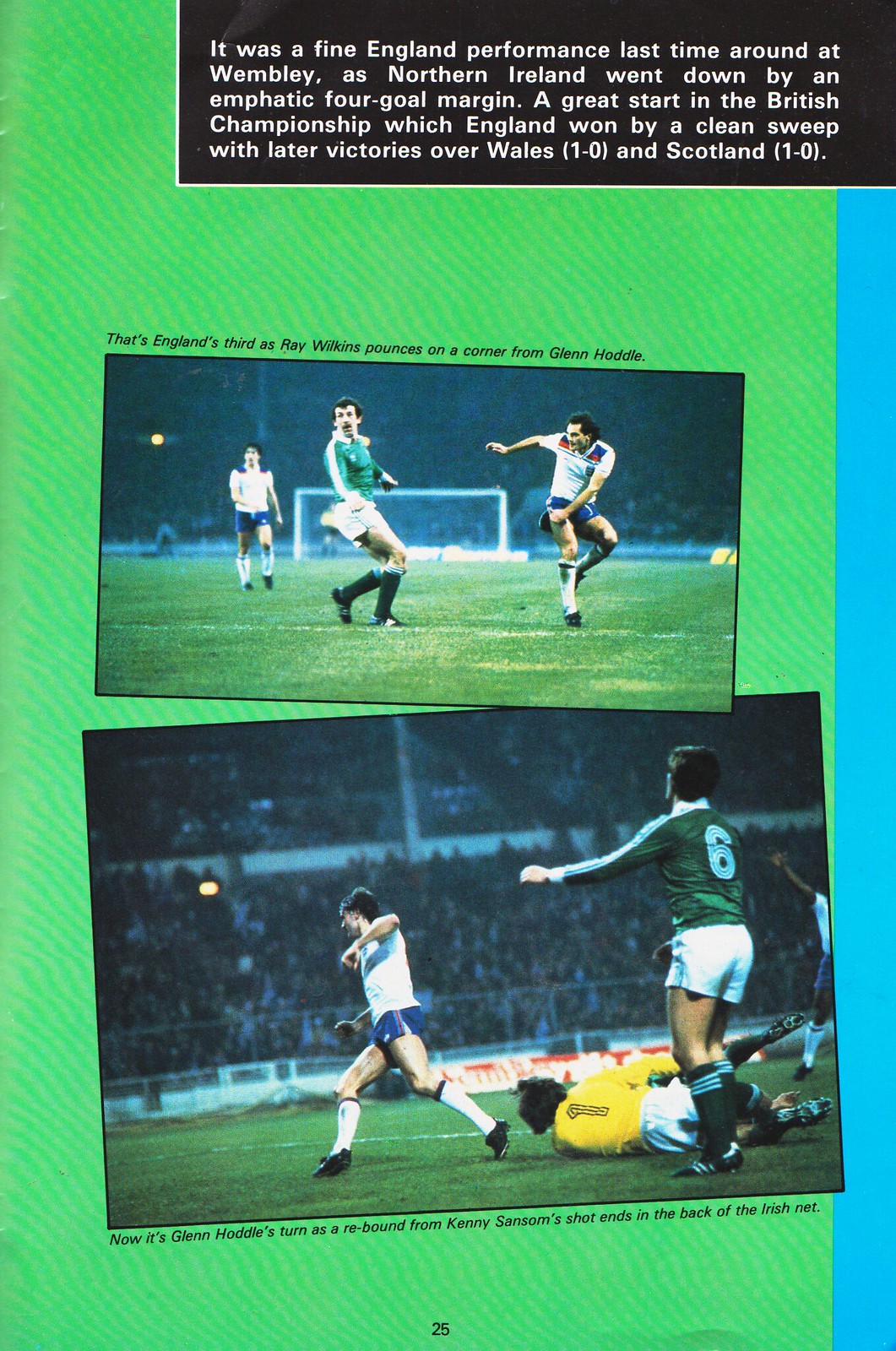The image is a colorful scan from a magazine or an official program page about a soccer game between England and Northern Ireland. The background is predominantly light green with dark green stripes and a thin blue border running down the right side. At the top of the page, there is a black box with white text detailing an emphatic England performance at Wembley, where Northern Ireland lost by a four-goal margin, contributing to England's clean sweep in the British Championship, including subsequent victories over Wales and Scotland.

Superimposed on the page are two angled photographs. The top, larger image shows three players on a green soccer field with a goal and stadium seating in the background. The scene captures England's third goal with Ray Wilkins in a white shirt pouncing on a corner from Glenn Hoddy. To his right is a player in a green shirt, and on the far right another player in a white shirt, all involved in the goal action.

The bottom, smaller photograph displays another match moment where Glenn Hoddy scores as a rebound from Kenny Sansom's shot ends up in the Irish net. The image includes a player in a white shirt running, a yellow-shirted goalkeeper numbered 1 on the ground, and another green-shirted player. The crowd is visible in the background, adding to the dynamic scene on the green field. The page is marked with the number 25 at the bottom.